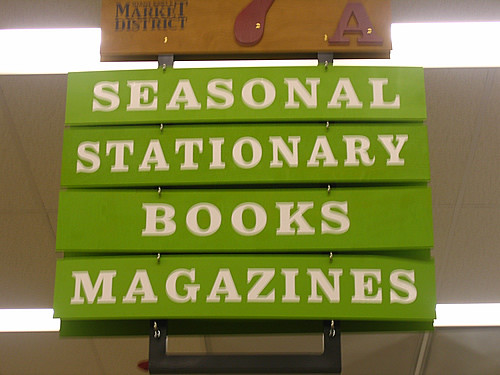The photograph appears to have been taken indoors in a store, capturing an upward view towards a brownish-colored ceiling with horizontal fluorescent lights spanning the width of the image. Dominant in the scene is a prominent wooden sign reading "Market District," with the letter "A" visible on the right side. Below this wooden sign, four narrow, lime green signs are attached by metal fasteners. Each of these green signs bears white capital letters, sequentially reading: "SEASONAL," "STATIONERY," "BOOKS," and "MAGAZINES." The signs create a cascading effect, prominently displayed against a light brown, paper-like background. Additionally, a rectangular red element can be seen among the signage, enhancing the organizational aesthetics of the store's interior.